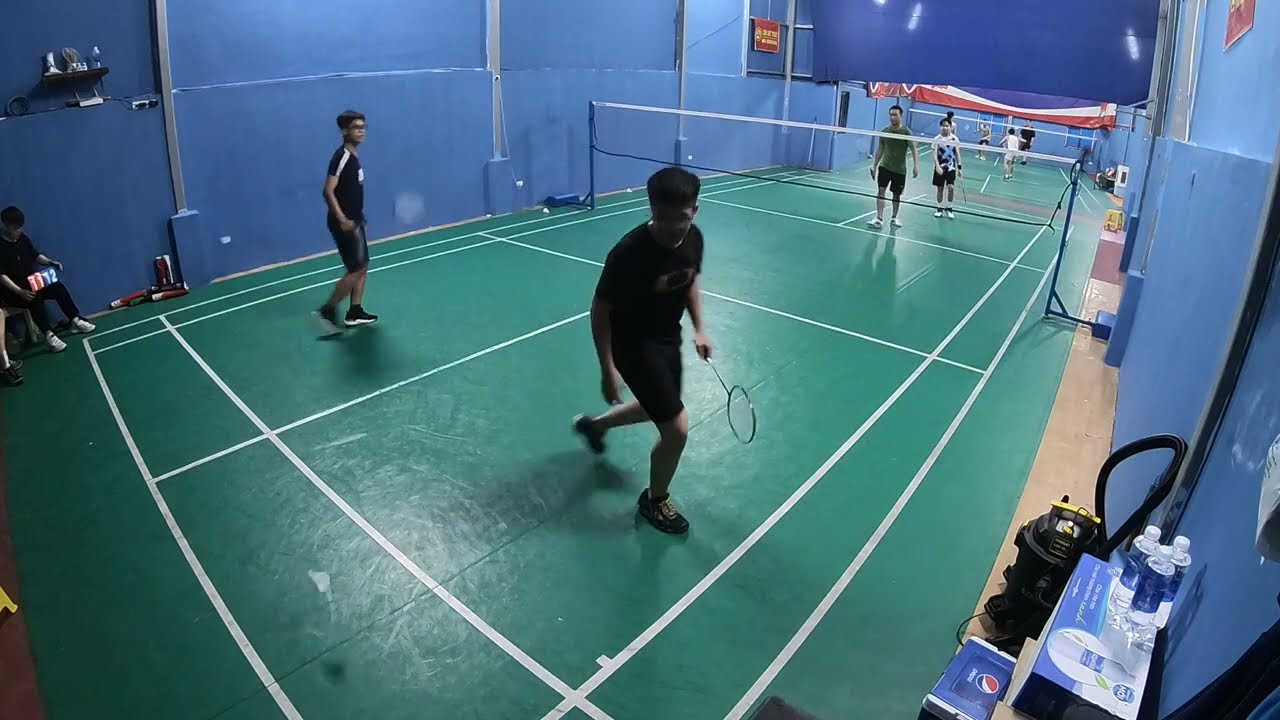The horizontally aligned rectangular image captures an indoor sports scene centered on a green court with white lines resembling a tennis or badminton court, but potentially used for racquetball or pickleball. The blurred action suggests a game in progress, with attention drawn to a preteen boy in the foreground, positioned slightly turned with a badminton racket in his left hand, and short hair. To his left stands another boy with short black hair and glasses, dressed entirely in black attire and obscured on his left side making it unclear if he holds a racket. 

In the mid-left corner, a person dressed in black, potentially a scorekeeper, holds a red and blue scoreboard with white numbers. The top right of the image shows two additional participants, one in a green short-sleeve shirt and black shorts, and another in a white patterned shirt, also with black shorts, both holding rackets, suggesting a doubles match. The background reveals a second similar court, marked by blue walls and a prominent red and white banner extending across the space. Additionally, the scene includes a table in the foreground with supplies such as water bottles and a box of Pepsi, indicating preparation for an event or tournament.